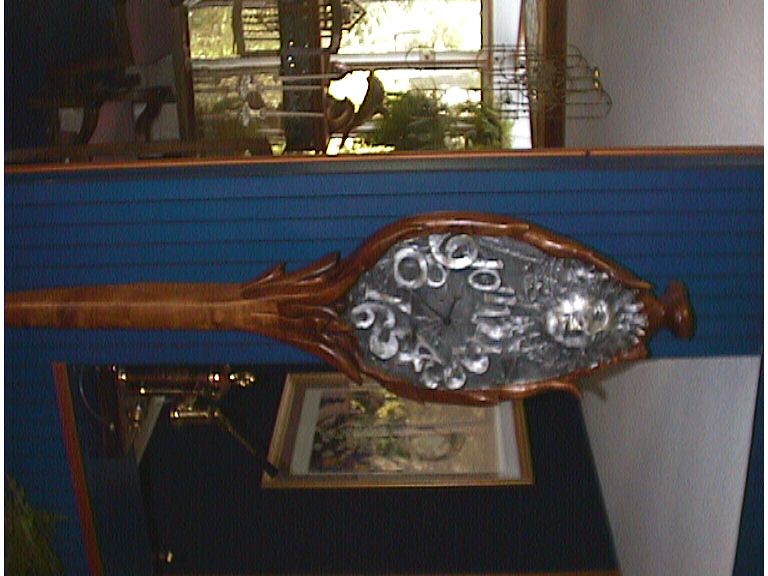This photograph captures an elegant, vintage-themed interior of a home. The viewer is provided a sideways perspective of the image, which prominently features an ornate stand-up clock positioned centrally. The clock boasts a tall, intricately carved wooden stand leading up to a teardrop-shaped wooden frame, richly adorned with elaborate crystal decorations. At the top of the clock, there is a detailed, metal sun with a face, below which lie the clock's numbers, arranged in an eccentric, haphazard circular pattern with each number varying in size. The black clock hands, though faintly visible, indicate a time of approximately 9:37 or 9:40.

The room exudes an antique charm with its blue wooden paneled walls, framed meticulously in wood, and its classic popcorn white ceiling. A large black wall hosts a grand golden-framed painting or artwork, which remains blurry and grainy in the photograph. Adding to the room's vintage ambiance, the interior is filled with numerous plants and metal ornaments suspended from the ceiling, alongside traditional, classical furniture pieces, all of which contribute to the nostalgic, cluttered atmosphere of what appears to be an older home.